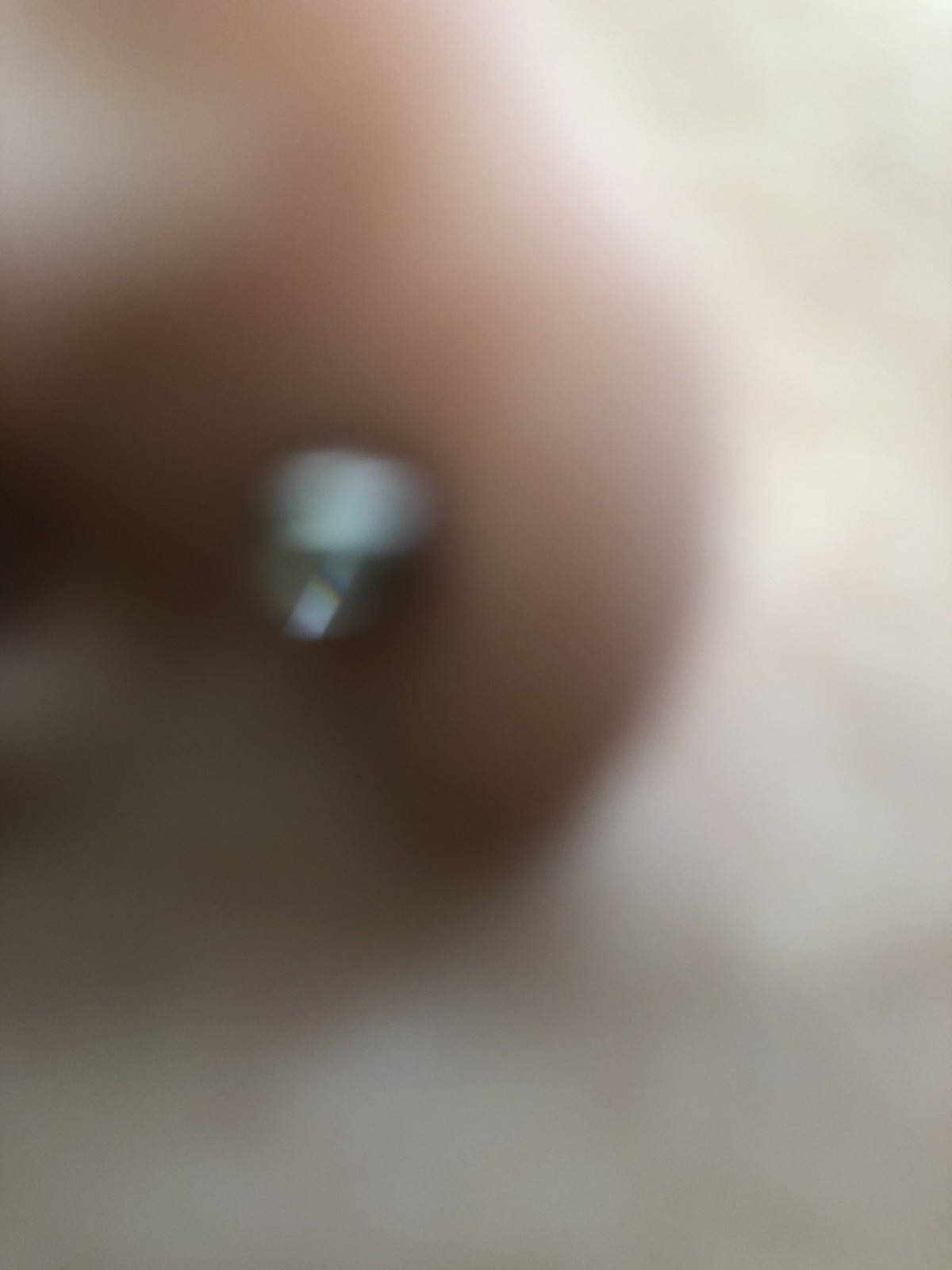This image is an extremely blurry, up-close photograph primarily in tan, peachy flesh tones with some light gray accents. It's difficult to discern the precise subject, but it appears to be a part of someone's face, likely the side of a nose, featuring a small, reflective silver or white stud, possibly a piercing. The stud is positioned about three-fifths up the image and two-thirds towards the left. The surrounding area includes shadows and light reflecting off the person's skin. The background remains indistinct, but consists of lighter beige and white areas, possibly indicating additional skin or fabric, and is generally lighter towards the upper right corner. Despite the intense blurriness, the prominent flesh tones and the presence of the small shiny object suggest that this is a close-up of a pierced nose or an earlobe with a stud earring.